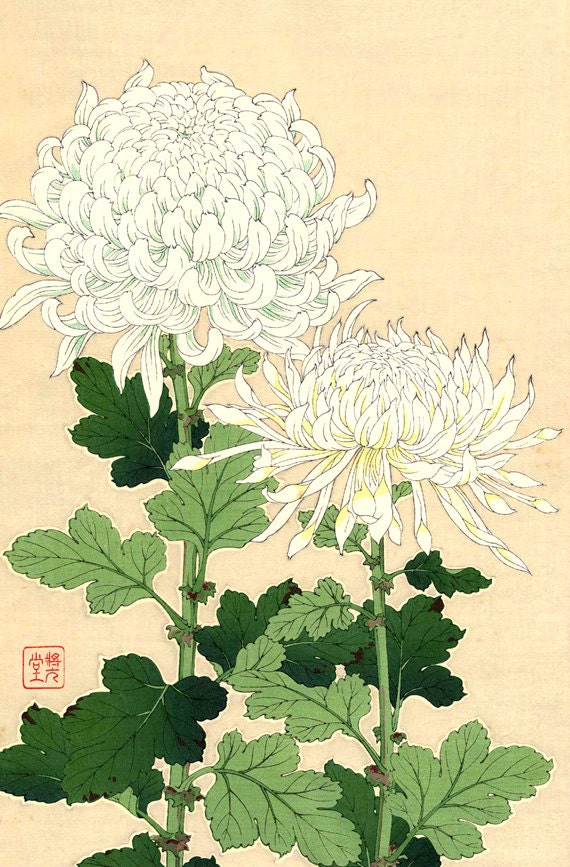This image depicts an Asian, possibly Japanese, drawing of two flowers on antique, off-white paper. Both flowers feature green stems and a mix of pale and dark green leaves. The flower on the left is taller with a thicker stem and larger, circular, bright white petals forming a bulb-like head. In contrast, the flower on the right is slightly shorter by the height of a full flower head and showcases more pointed, thin-tipped petals that have a whitish-yellow tinge. Its outer petals are beginning to fall, revealing yellow at their base and brown sections where the leaves join the stem. Additionally, a small, thin red square containing two or three Asian characters is positioned to the lower left of the taller flower.